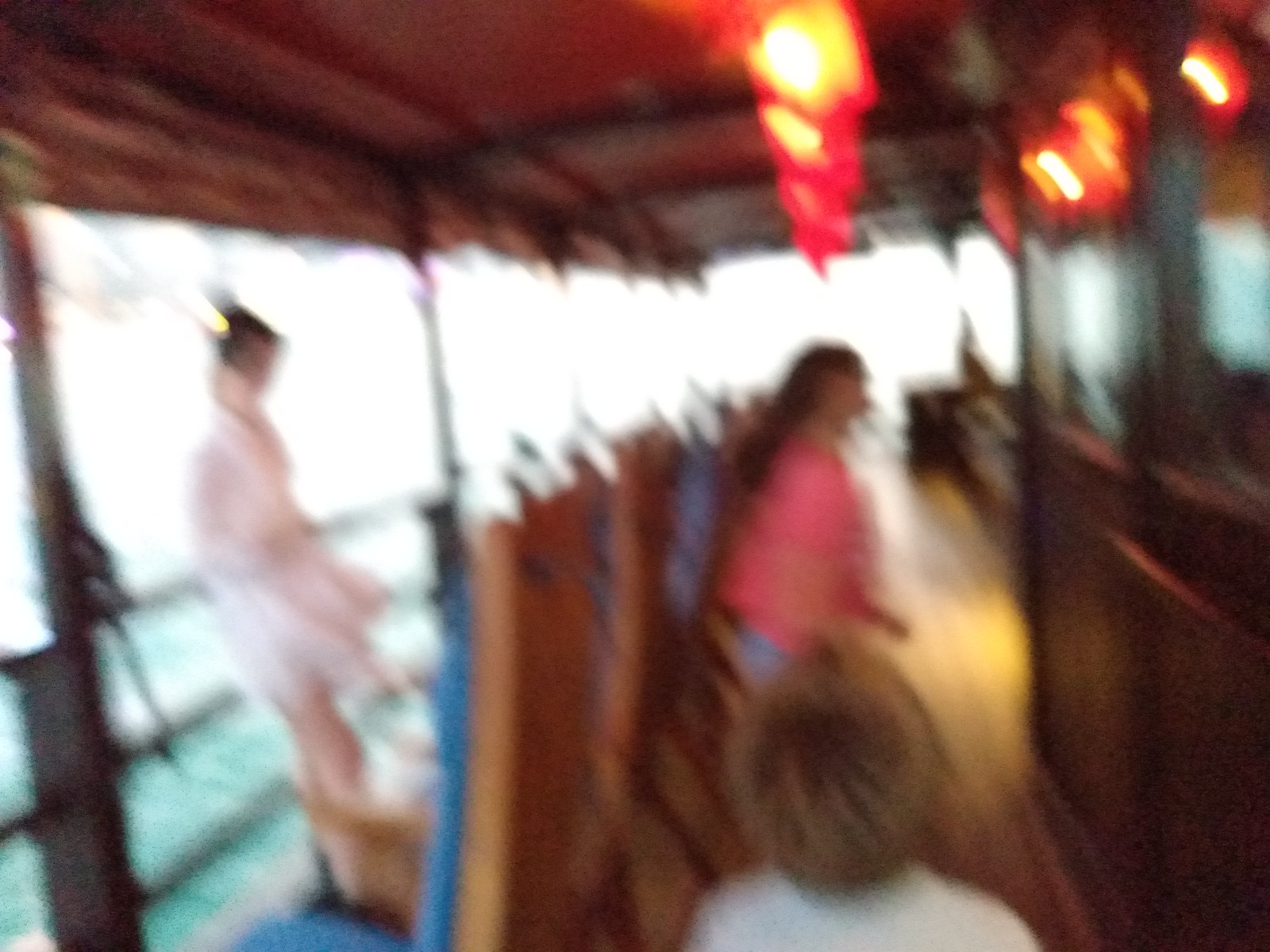A very blurred image captures a scene likely set on a boat or a roofed deck next to water. The background is an intense, pure white, as if illuminated by a bright flash, obscuring any sky or distant views. To the left, the railings of the boat are visible, beside a sea of vibrant aquamarine blue. Amidst the scene, under a canopy roof adorned with orange and red lighting, various elements of the deck come into focus, including brown wooden walls, floors, and large wooden chairs with blue cushions aligned near the railings. 

Against the railing, a woman in a floaty pink dress stands, seemingly nestled within a cardboard box-like structure. Nearby, another woman with long brown hair wears a pink shirt, and a small boy in a white shirt with short blonde or brown hair stands below her. The detailed setup, showing the intricate layout of wooden barriers and railings, enhances the scene set on the top deck of a boat or a similar structure encased in warm, brown hues.